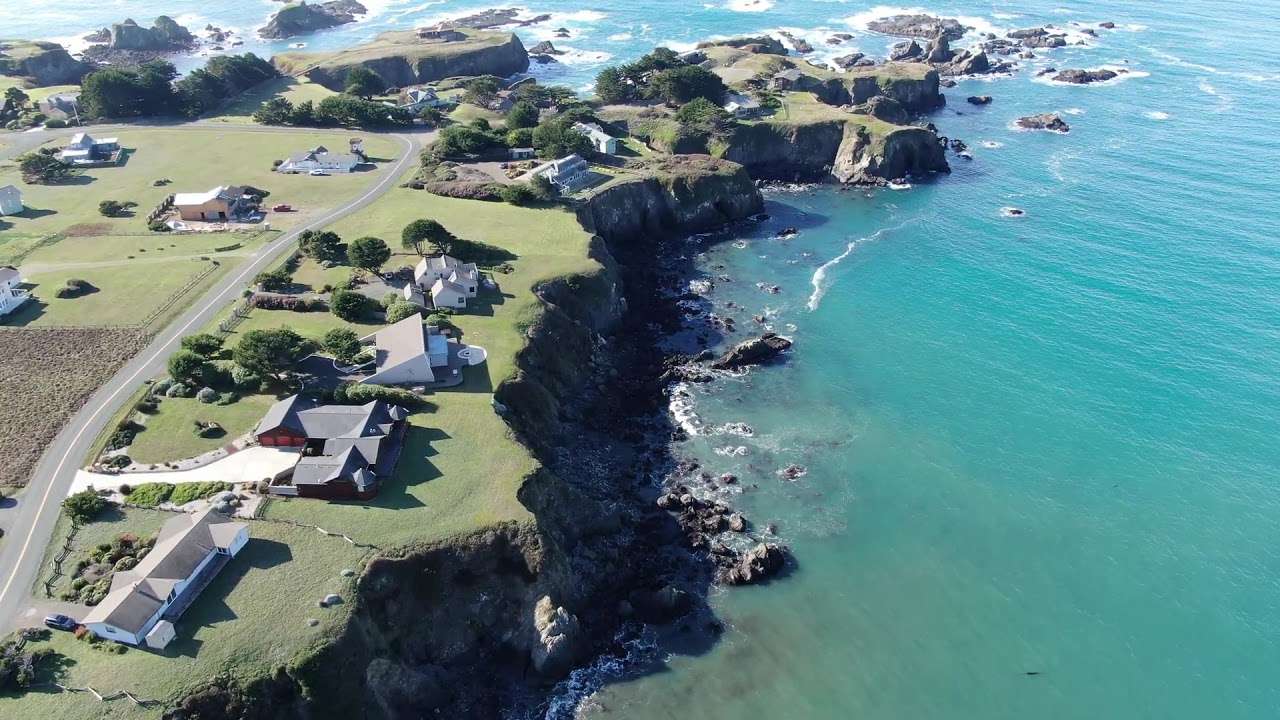The image is an aerial shot, likely captured from a drone or helicopter, showcasing an oceanfront town characterized by its dramatic cliffside setting. On the left side of the image, there are approximately seven to eight modern-looking houses, including a notable house with a grey roof and red sides, estimated to be around 2,500 square feet. The houses, separated by a road, vary in color and have unique driveways, with the surrounding area featuring lush greenery, trees, and grass. The right side of the image displays a turquoise, light bluish-green ocean with waves crashing against a rocky shoreline that extends from the center bottom to the very middle of the image. The homes are perched atop a rock formation or island, with the cliffside plunging roughly 30 feet down to the ocean. The entire scene exudes a harmonious blend of natural beauty with modern architecture, set against the vibrant backdrop of the deep blue ocean and rich green landscape.